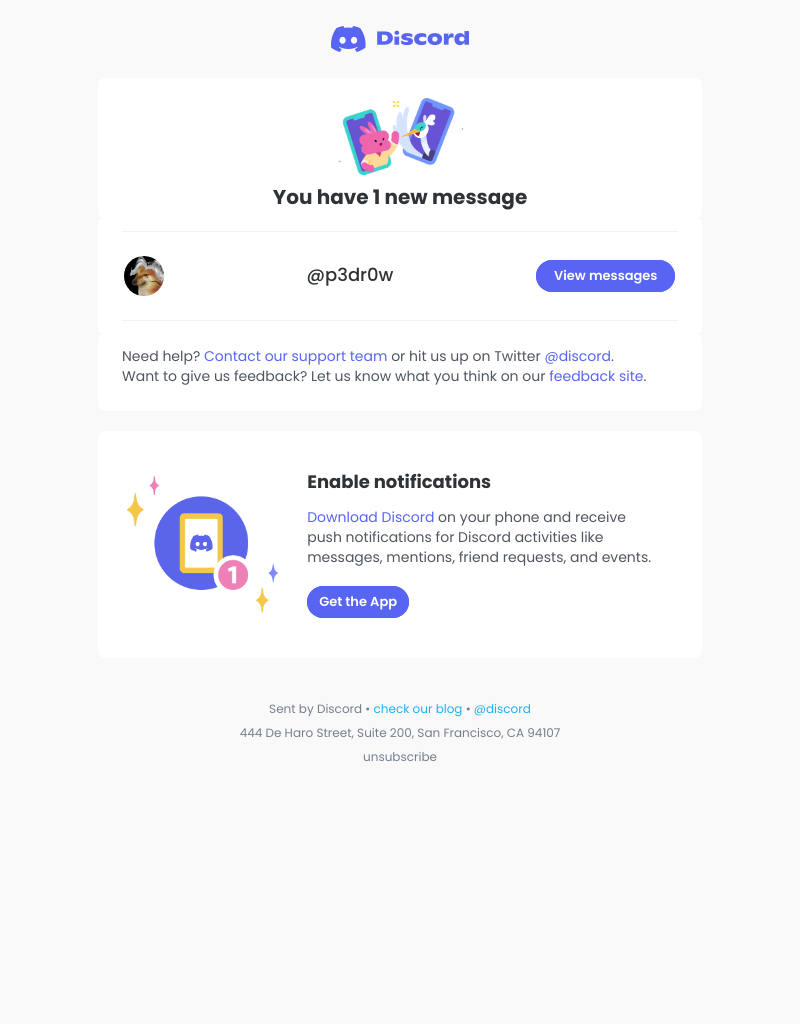The image can be described with the following detailed caption:

---

At the top of the image, there is a blue gaming controller icon, which is prominently displayed next to the word "Discord" in matching blue text. Beneath this header, two cell phones are visually showcased. The phone on the left features a pink character wearing a yellow shirt, depicted in a dynamic, 3D manner as if emerging from the screen. The phone on the right displays a blue screen with a white character illustration.

Below these phone images, black text reads, "You have one new message." To the left of this message, there is a small circle designated for a profile picture, while to the right, the text "@P3DR0W" is displayed, followed by a blue rectangular button labeled "View Messages."

The next section features a blue circular icon with a game controller inside it. A red circle with the number "1" is positioned in the upper right corner of this icon, and yellow retro starbursts embellish the top and lower right corners of the circle. To the right of this icon, text reads, "Enable Notifications." Beneath this, in blue text, it says, "Download Discord" followed by explanatory text: "on your phone and receive push notifications for Discord activities like messages, mentions, friend requests, and events."

Finally, at the bottom of the image, within a blue circle, white text encourages action with the phrase, "Get the App."

---